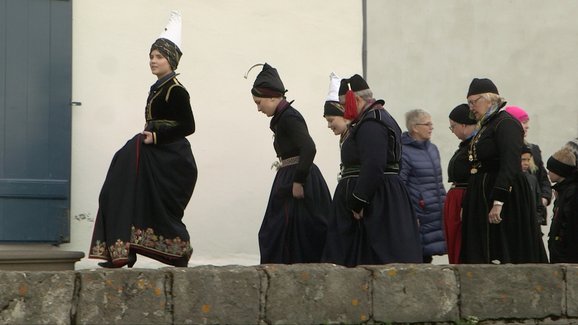A procession of five people in traditional Euro-Asian attire ascends a set of stone steps partially hidden behind a row of bricks in the foreground. The group consists of three women at the front followed by two men, all dressed in long, dark-colored robes with ornamental trims. The women's headdresses vary, with one donning a black hat topped with white, and another featuring a black hat with a curved white piece. The man in the middle wears a red, tasselled hat. The background reveals a cold, wintery setting with women, children, and older individuals clad in jackets, suggesting they are outside a building, possibly a church with a big blue door and a grey doorway. An elderly woman with white hair and glasses watches the scene while a person in a bright pink hat and several children add subtle touches of color to the backdrop. The woman leading the procession lifts her thick dress as she gazes into the distance, embodying a sense of cultural tradition and solemnity.